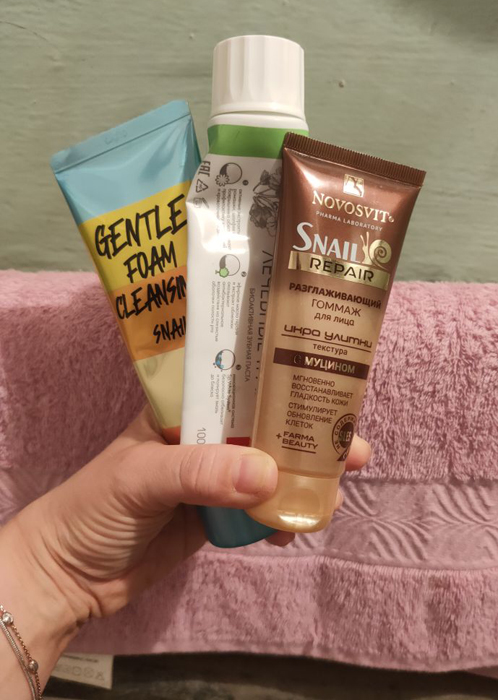In the image, taken in a bathroom setting, a pink hand towel with a ruched pattern is visible in the background. The focus is on a left hand adorned with a silver bracelet and a chain-like silver bracelet featuring large silver beads. This hand is holding three products. The top product, situated on the right side, is labeled "Novosvit Pharma Laboratory" in gold text, followed by "Snail Repair" and an illustration of a snail. Below this text, there are additional writings in an unknown language, though phrases like "PLUS Farma Beauty" are discernible. The middle product resembles a toothpaste tube with an oversized cap, but no English text is legible. The tube is white with a green stripe at the top. The bottom product, another squeezy tube similar to those used for conditioners, displays the text "Gentle Foam Cleansing Snail." This tube is decorated with multiple colored stripes.